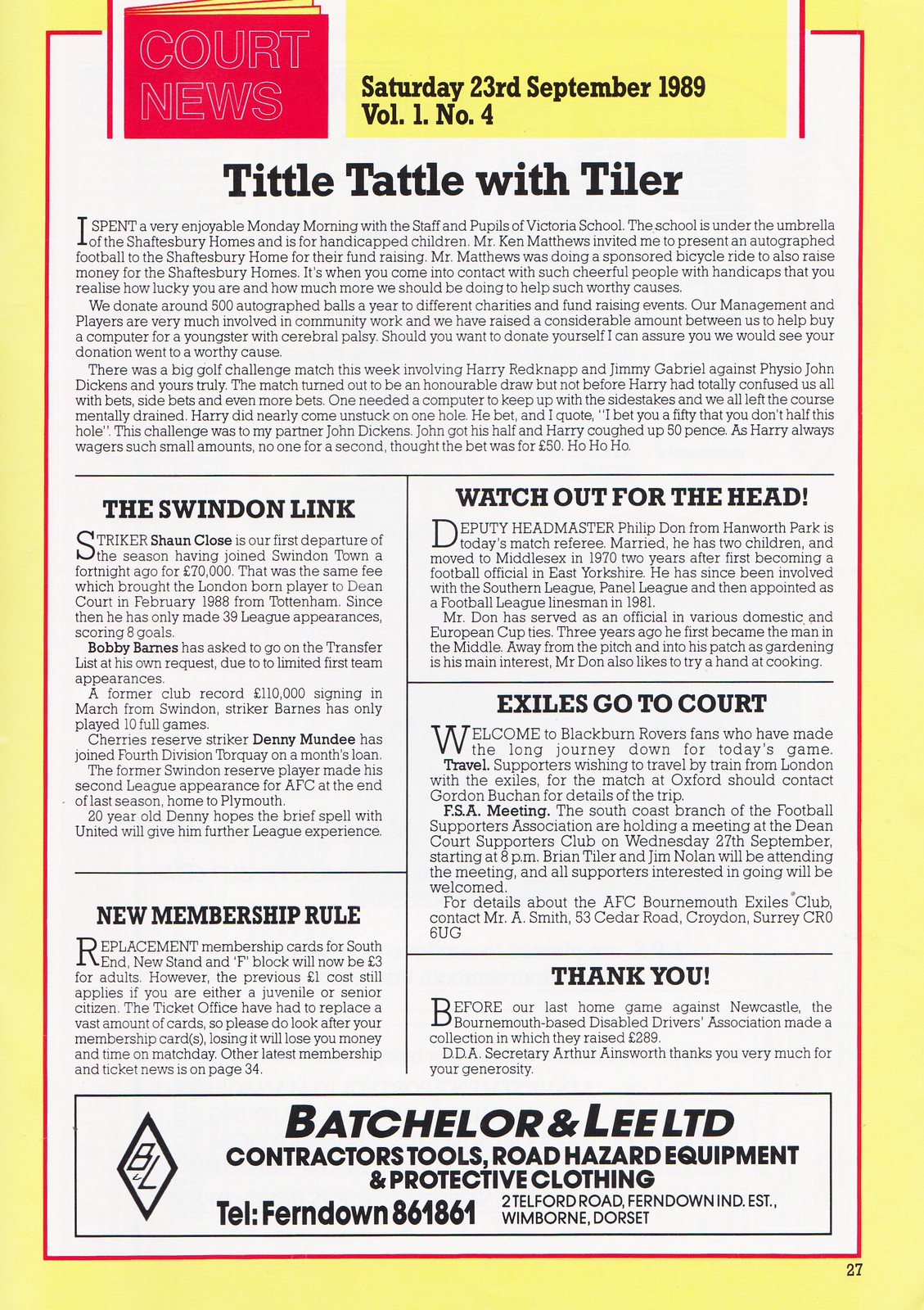The image is a page from a magazine or newsletter with a predominant yellow background and a white rectangular center bordered by a narrow red line. At the top, there is a red box containing the title "Court News" in white lettering. Adjacent to this title, in black text within a yellow box, it reads "Saturday, 23rd September 1989, Volume 1, Number 4."

The white central area is divided into several sections with different article titles, though the text is too small to read in detail. The articles are titled "Tittle Tattle with Tyler," "The Swindon Link," "New Membership Rule," "Watch Out for the Head," "Exiles Go to Court," and "Thank You."

The bottom portion of the page features an advertisement on a white background. It includes black text that reads, "Batchelor and Lee LTD, Contractor Tools, Road Hazard Equipment, and Protective Clothing," followed by the contact information: "Telephone Ferndown 861861, 2 Telford Road, Ferndown IND, Established Windbourne Dorset."